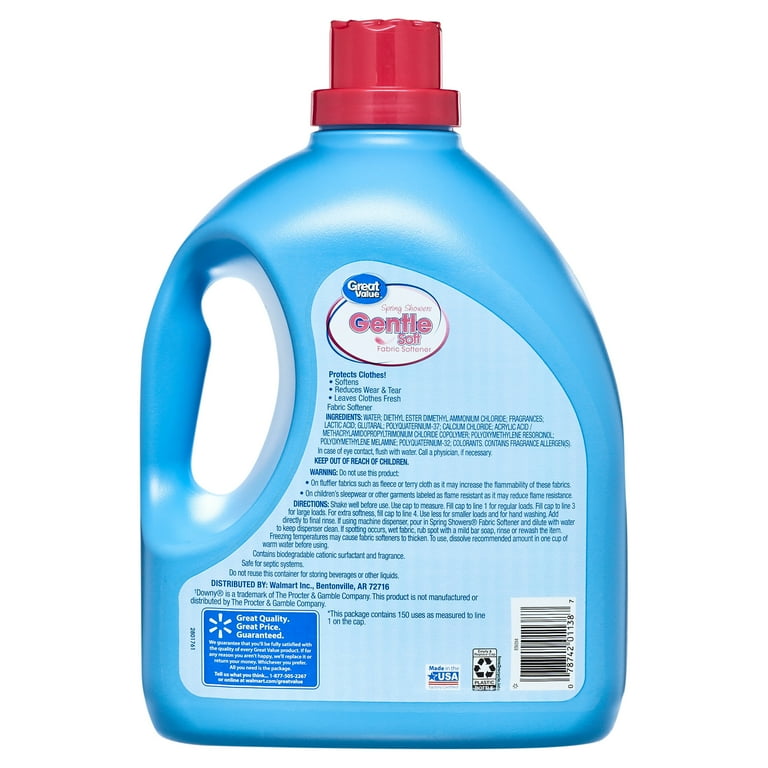This is a product photograph of the back side of a Great Value Spring Shower Scented Gentle Soft Fabric Softener bottle. The bottle is made of light blue plastic and features a bright red cap for easy identification. An ergonomic handle is integrated into the left side of the bottle for convenient carrying and pouring. The label on the back is primarily a lighter blue color and provides various details. At the top of the label is the Great Value Spring Shower Gentle Soft Fabric Softener logo. Below the logo, the label contains practical information such as ingredients, usage directions, and safety warnings. On the bottom left of the label, there is a Walmart Guarantee stating "Great Quality, Great Price, Guaranteed," adjacent to a "Made in the USA" logo, a recycling logo, and a large rectangular barcode. The bottle appears to hold approximately one gallon of fabric softener.